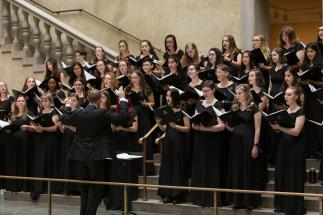The image depicts a large choir, predominantly composed of women dressed in black dresses, holding black folders with white sheet music. They are arranged in four rows on stone risers, facing a conductor who stands in front of them with his hands raised, conducting the ensemble. The conductor, attired in a black suit, stands before a podium that also holds sheet music. Behind the choir is a light gray, marbled stone wall, with a similarly colored staircase curving upwards to the left. The setting suggests a formal performance space designed to highlight the choir’s arrangement and acoustics.